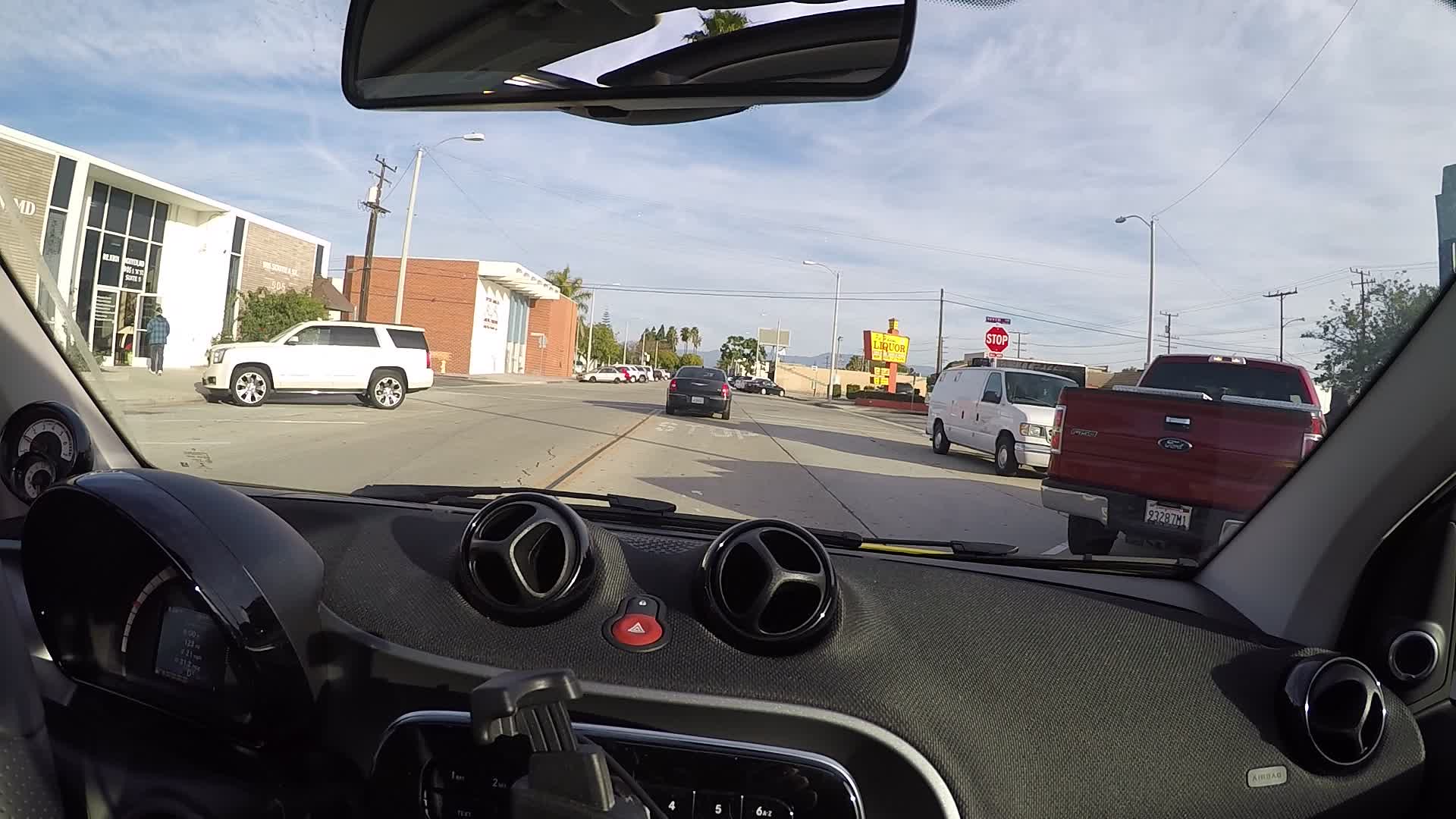This photograph, captured from the passenger side of a modern vehicle with a black interior, portrays a street scene through the windshield and over the dashboard. Prominently displayed are the vehicle's dashboard gauges and a rearview mirror positioned at the top of the image. The car is moving along a light gray asphalt road, heading toward a stop sign. Ahead, a black car is visible in the foreground, preparing to stop. On the right side of the image, a red truck, possibly with a California license plate, is parked, drawing attention along with a large yellow liquor store sign that's quite noticeable against the skyline. To the left, a white SUV is also parked near a nondescript, single-story brick building with a glass-front entrance featuring large windows and a door. In the background, you can glimpse some mountains, palm trees, and other types of trees, suggesting a west coast location. White clouds dot the sky with patches of blue peeking through.